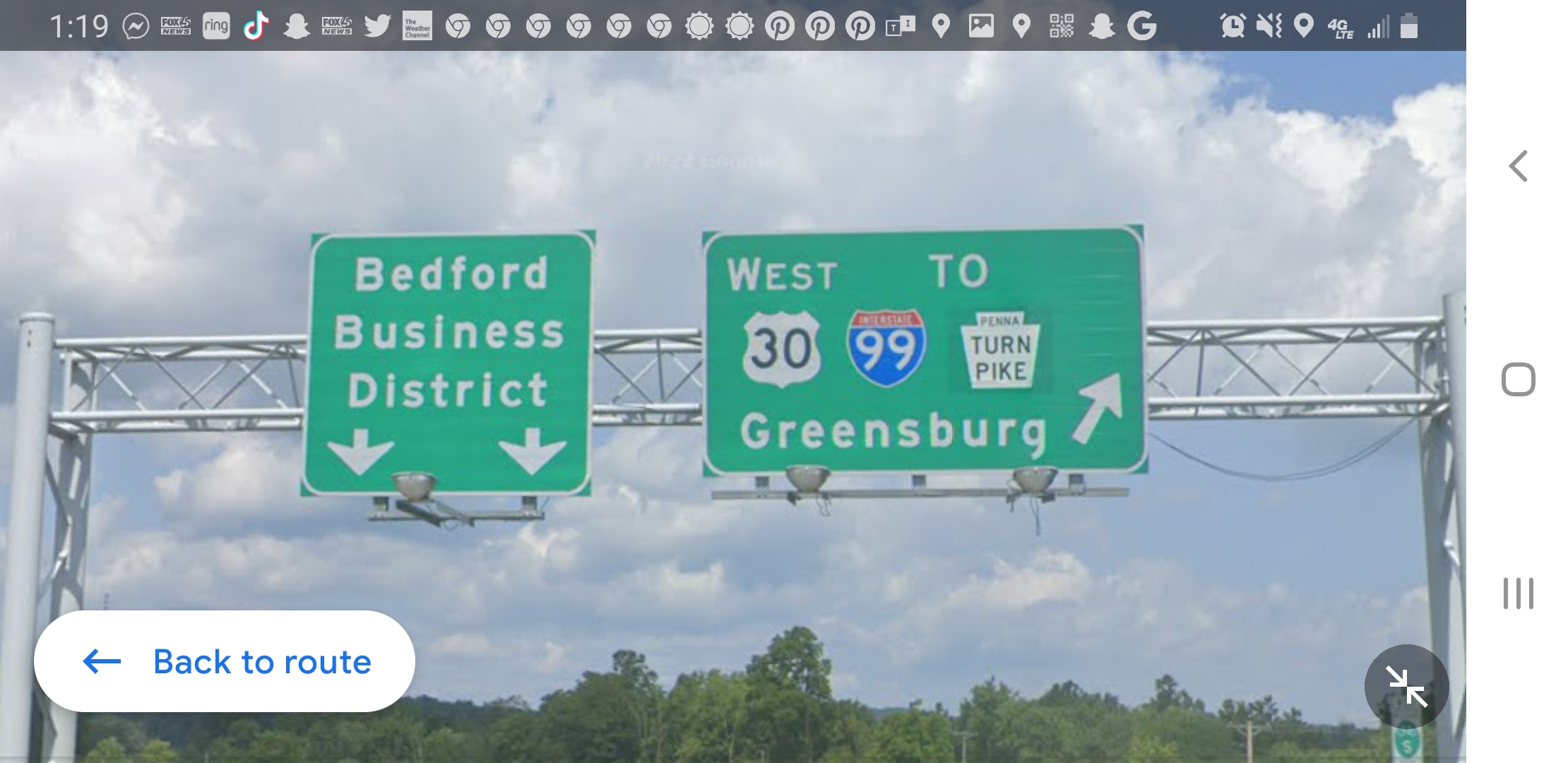This is a detailed screenshot captured on a smartphone. The top of the image displays various icons in white on a black background, typical of a phone's status bar. The time is shown as 1:19, and there are icons for Messenger, TikTok, Twitter, and several notifications from Chrome, Pinterest, and a weather app. Additionally, the battery level and signal bars are visible.

The main focus of the screenshot seems to be a portion of Google Maps. In the lower-left corner is a rectangular logo reading "Back to Route" in blue with a left-facing arrow of the same color, indicative of an option to return to the original navigation path.

Central to the image are two highway signs. The sign on the left is square and green, featuring the text "Bedford Business District" in white letters, with two arrows pointing downward. Adjacent to this is a more rectangular highway sign displaying "West to 3099 and Turnpike, Greensburg" with an arrow pointing diagonally to the right. The background reveals a scenic view, showing a sky dotted with fluffy white clouds and a line of green trees along the horizon.